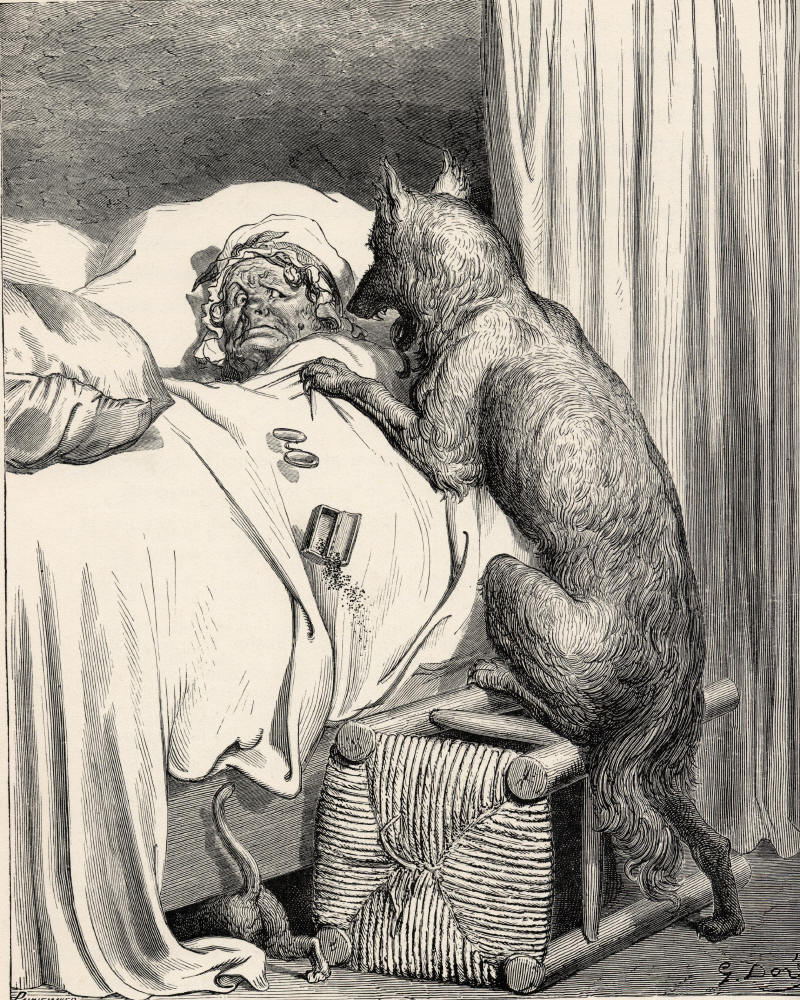This intricate pencil and ink drawing, resembling an 1800s cartoon lithograph, depicts a dramatic bedroom scene. At the center lies an older woman, her frightened expression framed by her cap and gown, as she gazes at a large dog or wolf that has leapt onto her bed, knocking over a stool below. The dog's detailed fur, meticulously rendered in pencil, conveys a sense of wild energy as its paws press against the bed sheets. Scattered across the floor are items including a pair of reading glasses and what appears to be a box spilling its contents. Adding to the chaos, a cat or possibly a rat is seen moving under the bed, with just its tail and back leg visible. The bed sheets cascade to the ground, revealing the dark backdrop and a curtain on the right, enhancing the sense of confinement and tension. The use of black and white contrasts sharply with the detailed textures, capturing the intense, almost cartoon-like essence of the scene.